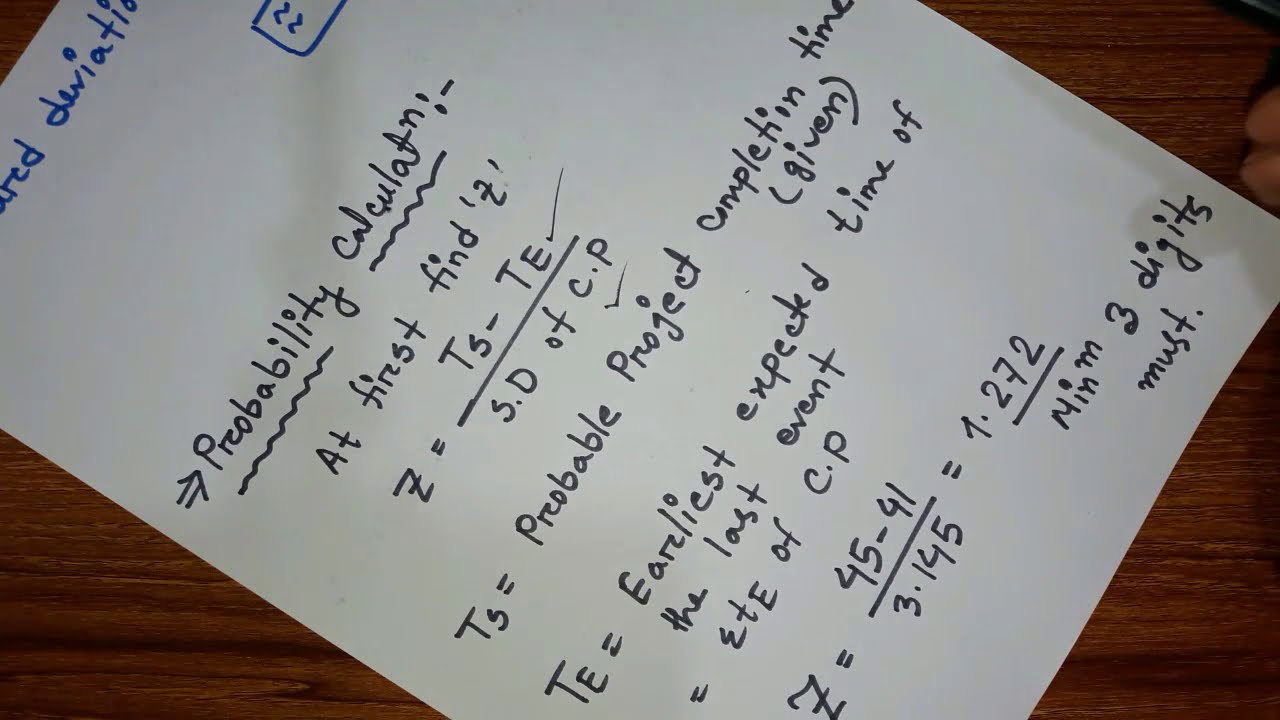This photograph captures a tilted white piece of paper lying diagonally to the left on a rich brown, dark wooden surface. The top left corner of the paper, which appears in the upper left section of the image, features blue writing. Below this, black handwriting reads "Probability Calculation," followed by an underlined section beginning with "At first find Z." The paper includes several equations and notes, with one particular formula relating to the probable project completion time marked as "T5 equals probable project completion time (given)." Further down the page, the text continues with additional equations, including one labeled "TE equals earliest expected time of the last event." The paper appears to be homework or notes from a math or engineering class, captured in detail against the contrasting wooden background.